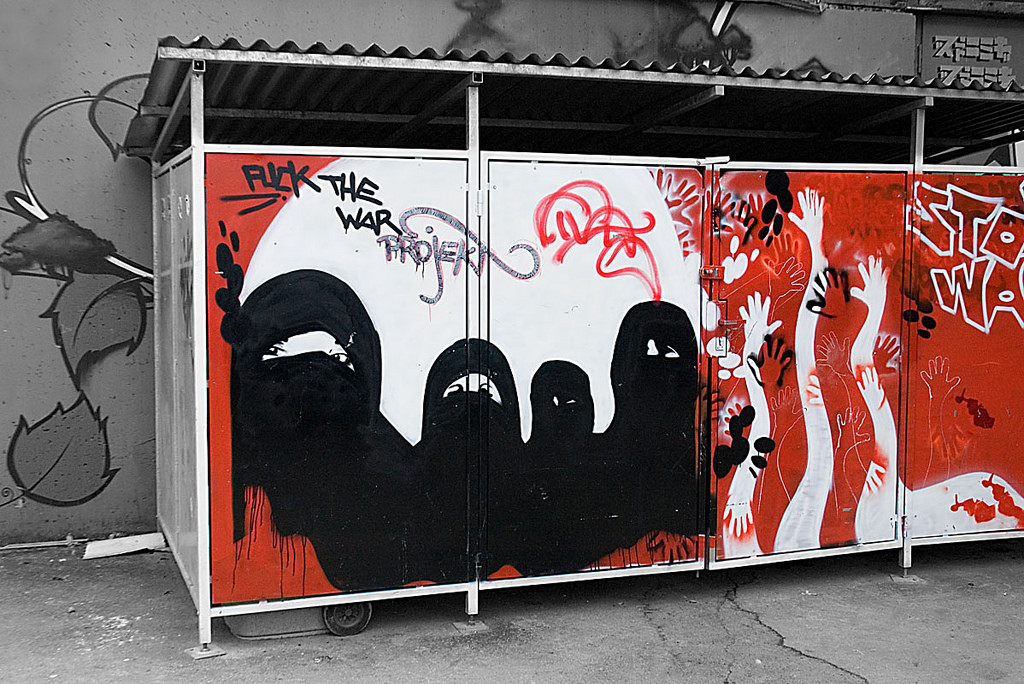This black-and-white photograph features a vividly colored graffiti art on an outdoor structure, likely a small metal building with a silver corrugated roof, situated on a concrete surface. The forefront depicts a trash receptacle holder adorned with striking red, black, and white artwork. On the left side of the graffiti are four women dressed in black niqabs and hijabs, only their eyes visible. A white circle, reminiscent of the sun, frames their heads, and above it, the phrase "Fuck the War Project" is emblazoned in black. To the right, white hands stretch upwards against a red backdrop, interspersed with red and white handprints. Beyond the hands, the white letters "Stop War" appear, though partly obscured. Additionally, the gray wall behind the structure features gray-painted leaves and East Asian characters. The detailed and dynamic art vividly stands out against the monochrome surroundings, encapsulating a powerful anti-war message.